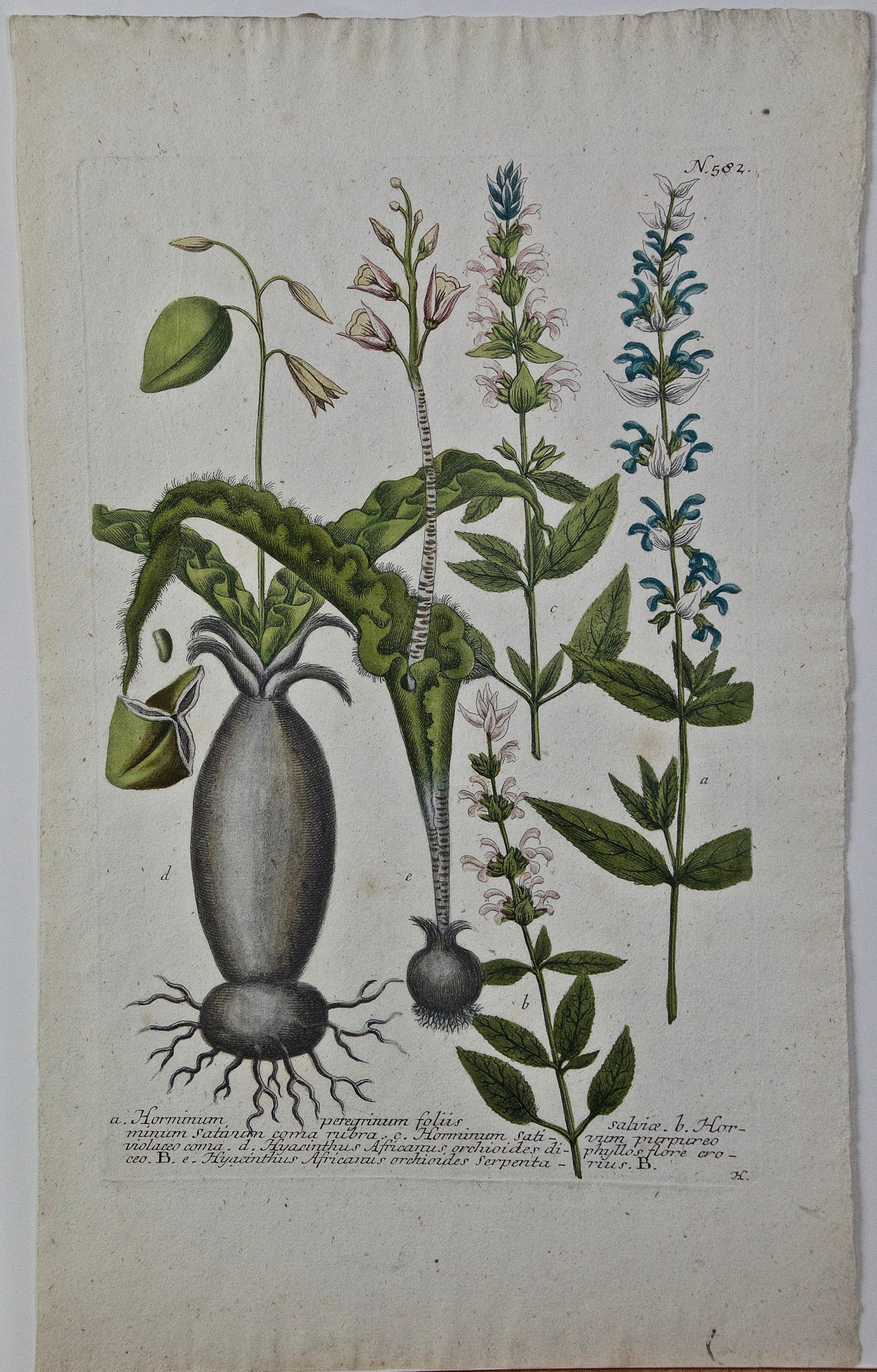This detailed vintage botany drawing, likely from the early 1900s, is rendered on a slightly crinkled, weathered piece of material that appears to be linen or canvas. The illustration features five different plants, with their detailed growth stages—from bulb to full bloom. The plant on the left showcases a gray bulb with green and pink leaves and flowers emerging from it, which appears similar to another centrally placed plant. Moving right, three additional plants are depicted; two feature blue flowers, while the central plant exhibits only stems, leaves, and pink flowers. The far-right plant displays a unique structure, almost resembling a Venus flytrap, but with leafier extensions. Below the botanical illustrations, there is cursive writing, possibly in a different language, which provides an explanation or labeling for the plants, though it's challenging to discern the exact language or meaning. The background is clear, and a number—502 or 582—is subtly visible in the backdrop, tying this historical piece to the study and appreciation of horticulture.